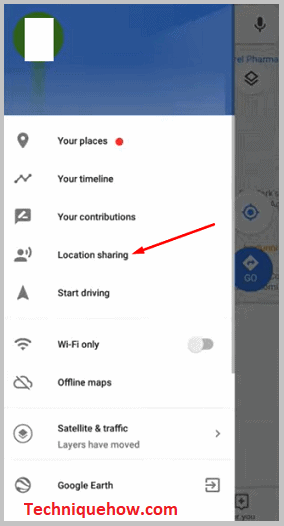In the image, there is a vertical rectangular layout dominated by elements related to navigation and maps. At the top, "techniquehow.com" is prominently displayed in red lettering. Below this, the top section features a blue background with a green hot air balloon icon that envelops a white square at its center. The background appears as a map interface, with a visible microphone icon on the right-hand side and a label marked "pharmacy."

Two circles are present, one white and one blue. The white circle contains a smaller blue circle, while the blue circle features a white diamond with the word "Go" inscribed within it. To the right of these circles is a long white rectangle that includes various labels such as "Your places" with a red dot beside it, "Your timeline" accompanied by a zigzag line, and "Your contributions."

"Location sharing" is marked with a red arrow pointing towards it, and an upward arrow indicates "Start driving." The "Wi-Fi only" option showcases a Wi-Fi signal icon next to it with a toggle switch. The "Offline maps" section is symbolized by a cloud crossed out with an "X" line, and "Satellite" and "Traffic" options are also mentioned.

There's a gray label indicating "Layers have moved," with a corresponding arrow pointing to the right. Following this, a circle with diamond shapes stacked on top of each other, where the top one is dark gray, introduces the "Google Earth" option. An adjacent arrow within a square outline points to the right, leading to further functionality.

Each element is arranged thoughtfully to facilitate easy navigation through the different options and settings related to map and location features.